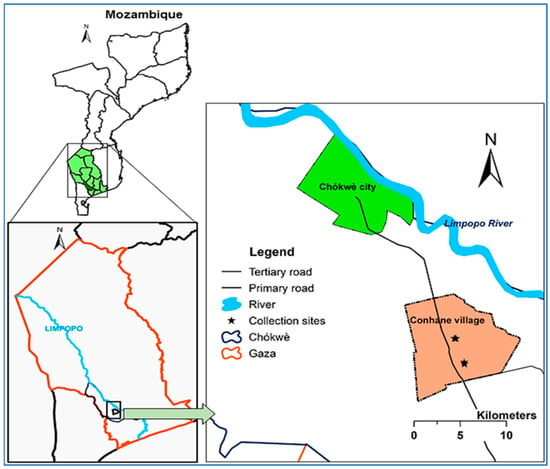This detailed vertical rectangular map, outlined in a thin blue line, prominently features the African country of Mozambique. The upper left corner of the map includes a black, drawn outline of Mozambique on a white background, with the country's name written in black text above it. The bottom part of this map section is shaded green. The map comprises multiple zoomed-in and enlarged sections for better detail. 

To the right, an orange-red line wraps around the central part, apparently depicting the Limpopo River, which is painted blue. A green-bordered box surrounds this river section, emphasizing "Chocui City" labeled within. Beneath this, another area is highlighted in pale orange, marked "Kanhane Village" and also referred to as "Cocaine Village" in the various captions. 

The map includes a legend on the left side, denoting symbols for roads, rivers, collection sites (marked by stars), and various other geographical details. The lower portion of the map shows additional areas like "Milano Village" and "Chippewa City," identified with green shading and pink colors respectively. Together, these elements provide a comprehensive and detailed visual representation of the respective locations in Mozambique.